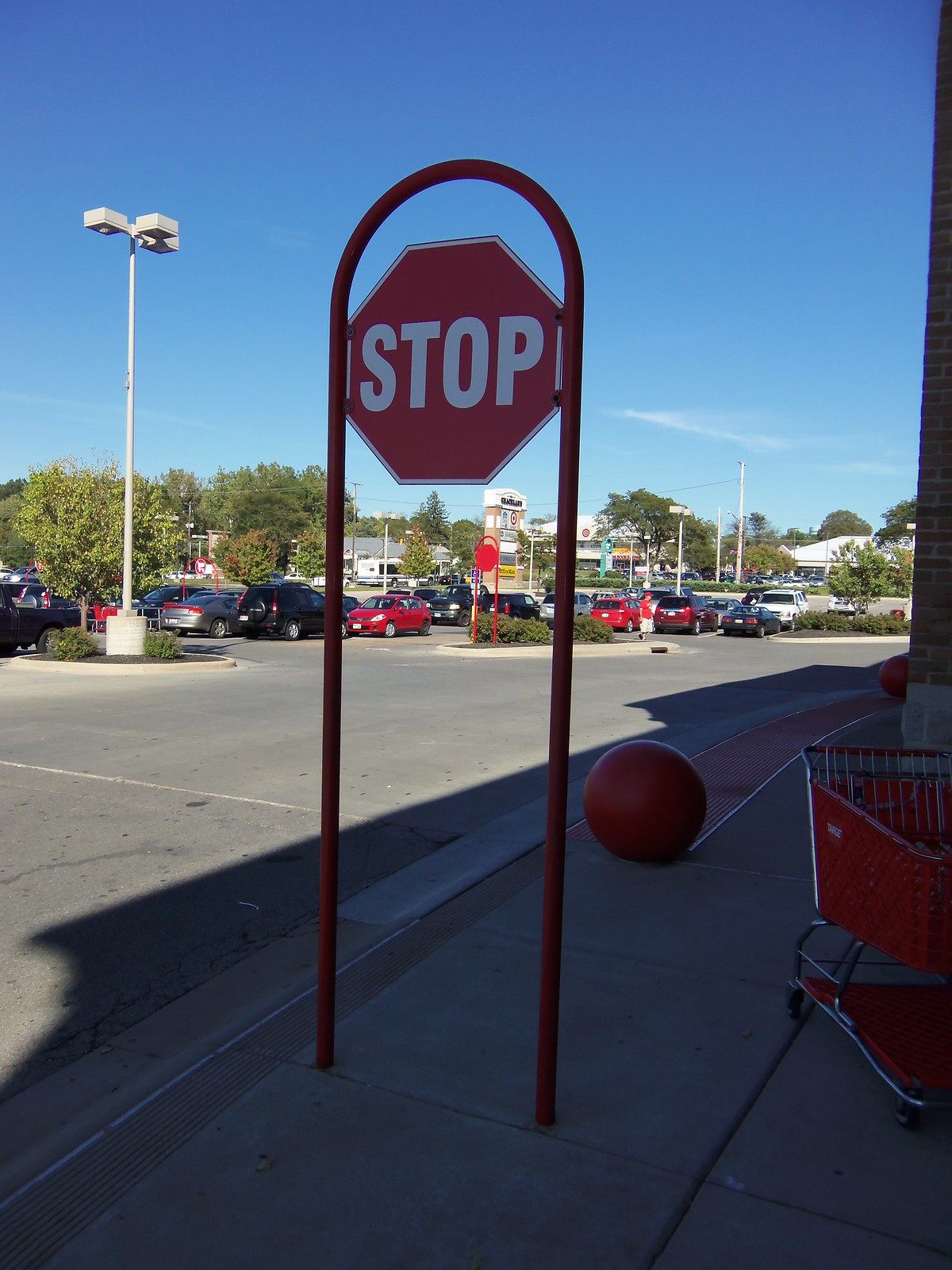This vertical rectangular photograph captures a sunny day in a Target parking lot, with a vibrant blue sky occupying nearly half the image, punctuated by a small white cloud on the right. Dominating the center is a stop sign, mounted uniquely on an upside-down U-shaped red metal frame, rather than a typical silver pole. The sign itself, shaded and slightly angled towards the lower left, displays the word "STOP" in bold white capital letters on a red octagonal background. To the right and partly off the lower left edge, a red shopping cart with a second layer and silver metal bars is visible. In the background, the parking lot stretches out with various cars in different colors like red, black, and silver. A tall ivory-colored lamppost stands near the top right. The scene features green trees and parts of other buildings, including the edge of the gray brick Target store and a possible gas station marked with a circular logo that could be 76. A signature red Target ball is on the ground behind the stop sign, reinforcing the retail setting. The photograph vividly showcases the mix of shaded and sunny areas created by the casting shadows from the Target building and other elements around the lot.